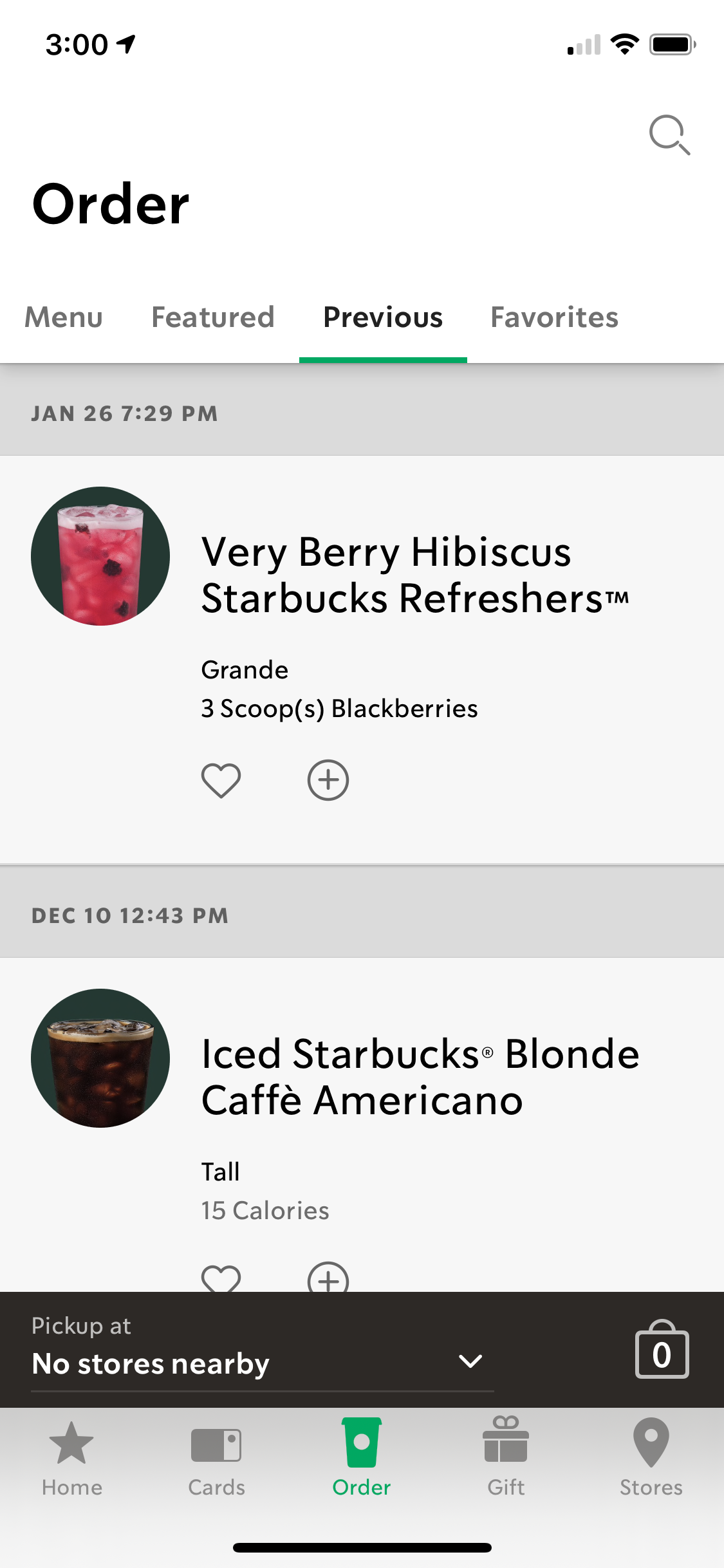The image depicts a phone screen showing the details of a previous Starbucks order in an application. At the top left corner, there's a status bar displaying the time "3:00" in black, followed by a directional arrow indicating compass navigation, and signal strength bars with only the first one lit up. Also visible are three Wi-Fi bars and a battery icon in black. 

Immediately below this status bar, there is a search icon represented by a magnifying glass on the gray background. Moving to the left, the word "Order" appears in black letters. Beneath this, there are four tabs named "Menu," "Featured," "Previous," and "Favorites." The "Previous" tab is highlighted in black with a green arrow indicating it is currently selected.

Under the tabs, there is a gray banner with the date "January 26th, 7:29 PM." Below this banner, a detailed section outlines a previously ordered item. There’s an image of a drink (a round circle with a glass containing pink liquid). To the right, the drink is identified as a "Very Berry Hibiscus Starbucks Refreshers™," specified as "Grande," with "3 scoops" of blackberries. Adjacent to this item is a heart icon and a gray circle with a plus symbol.

Following this item, another gray banner appears with the date "December 10th, 12:43 PM." Below this, there is a smaller, darker image that is difficult to distinguish. Beside it, the text describes an "Iced Starbucks Blonde Café Americano, Tall," noted to have "15 calories." This section also includes a white heart symbol and a white circle with a plus sign. 

At the bottom of the screen, a black banner states "Pick up at," followed by the text "No stores nearby" in white. To the far right of this text, a down arrow and a shopping bag icon with a white zero are displayed. The footer of the screen features navigation icons labeled from left to right: "Home" (with a star), "Cards" (with a tag icon), "Order" (with a green bin), "Gift" (with a wrapped gift icon), and "Stores" (with a map icon).